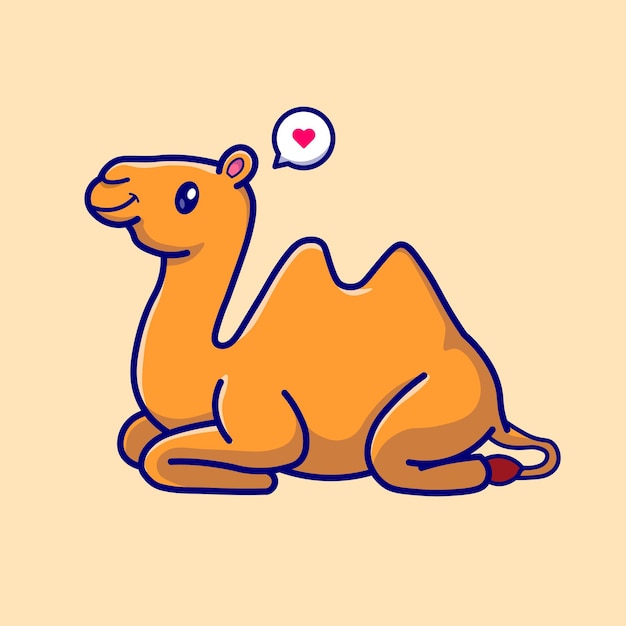The image is a square-format, juvenile-style illustration of a camel. The background is a gradient that shifts from pale orange at the top to a muted pink at the bottom. The camel, depicted in a side profile, is laying on its belly with its legs folded underneath and its neck straight up, giving a smiling expression with a large, cartoon-styled eye. The camel is primarily a light brown or tan color, with darker brown shadows for depth and dark blue outlining its entire form. Notable color details include a red tip on its curled tail and pink inside its ears. Just to the right of the camel's head, there's a small speech bubble with a white center and a red heart symbol inside. The cheerful and whimsical design of this illustration resembles the kind typically seen in greeting cards or emoticons.